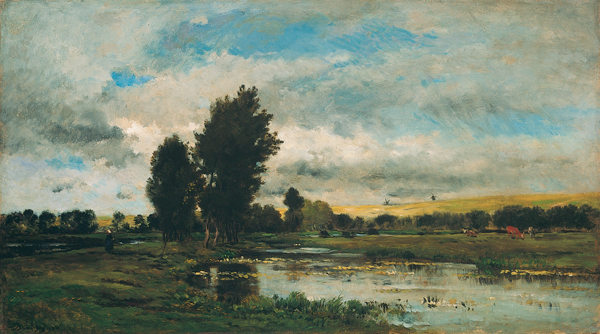The landscape painting, horizontally oriented, depicts a picturesque outdoor scene characterized by a reflective lake adorned with lilies in the immediate foreground, occupying mostly the bottom right part of the image. The lake's surface reflects light and shadows from the clouds above. To the bottom left, a grassy meadow shoreline leads to a line of trees along the horizon, with two prominent trees standing slightly to the right. The sky above is a vibrant blue interspersed with an abundance of white clouds. On the right side of the horizon, shorter trees and a hillside dominate the view, where indistinct figures or structures are visible, suggesting either people or buildings. At the right background of the painting, animals can be seen grazing. The entire scene, evocative of realism due to its lifelike detail, might even include a woman in a white headdress and black dress standing on the left bank, contributing to the serene and bucolic charm of the overall composition.